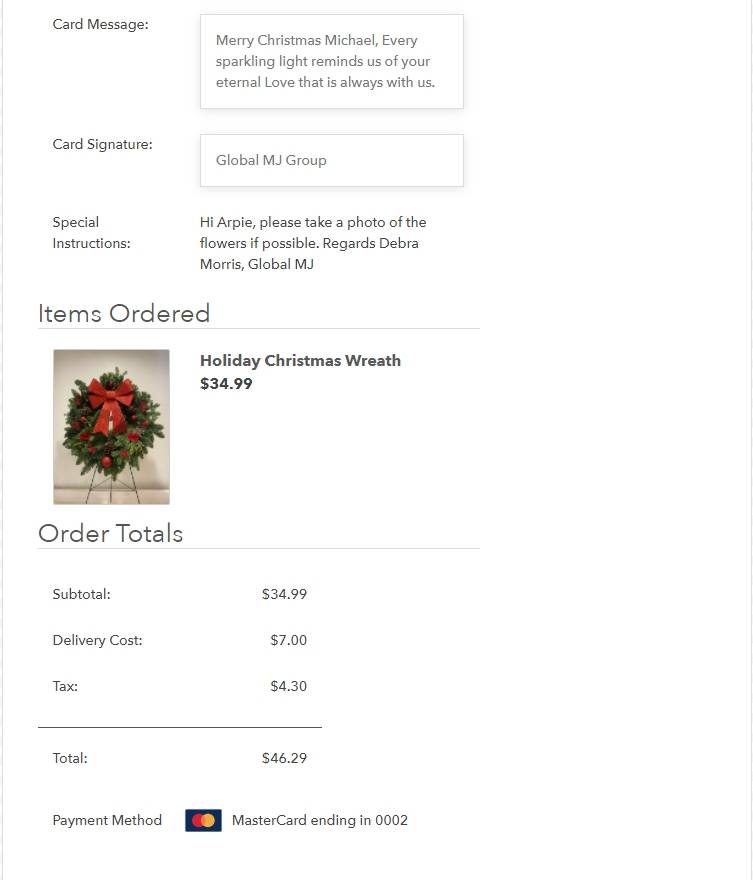This is a detailed screenshot of an order confirmation on a computer or mobile device screen.

At the top, a rectangular section with a white background displays "Card Message." To the right, there is a text box containing the message: "Merry Christmas, Michael. Every sparkling light reminds us of your eternal love that is always with us." Right below, another section labeled "Card Signature" has a box that states: "Global MJ Group."

Following this, there is a section titled "Special Instructions." The accompanying text reads: "Hi, ARPL. Please take a photo of the flowers if possible. Regards, Deborah Morris, Global MJ."

Subsequently, the "Items Ordered" section includes an image of a wreath adorned with a red ribbon, positioned on a stand. The description to the right of the image identifies the item as a "Holiday Christmas Wreath" priced at $34.99.

Below the image and the item description, there is an "Order Totals" section which lists the charges: a subtotal of $34.99, a delivery cost of $7, and tax amounting to $4.30. Below these, a line separates the summation from the final amount, which is stated as $46.29.

At the bottom of the screen, under the "Payment Method" section, there is an icon of a credit card displaying the familiar red and yellow circles of a MasterCard. The text indicates the card used is a MasterCard ending in 0002.